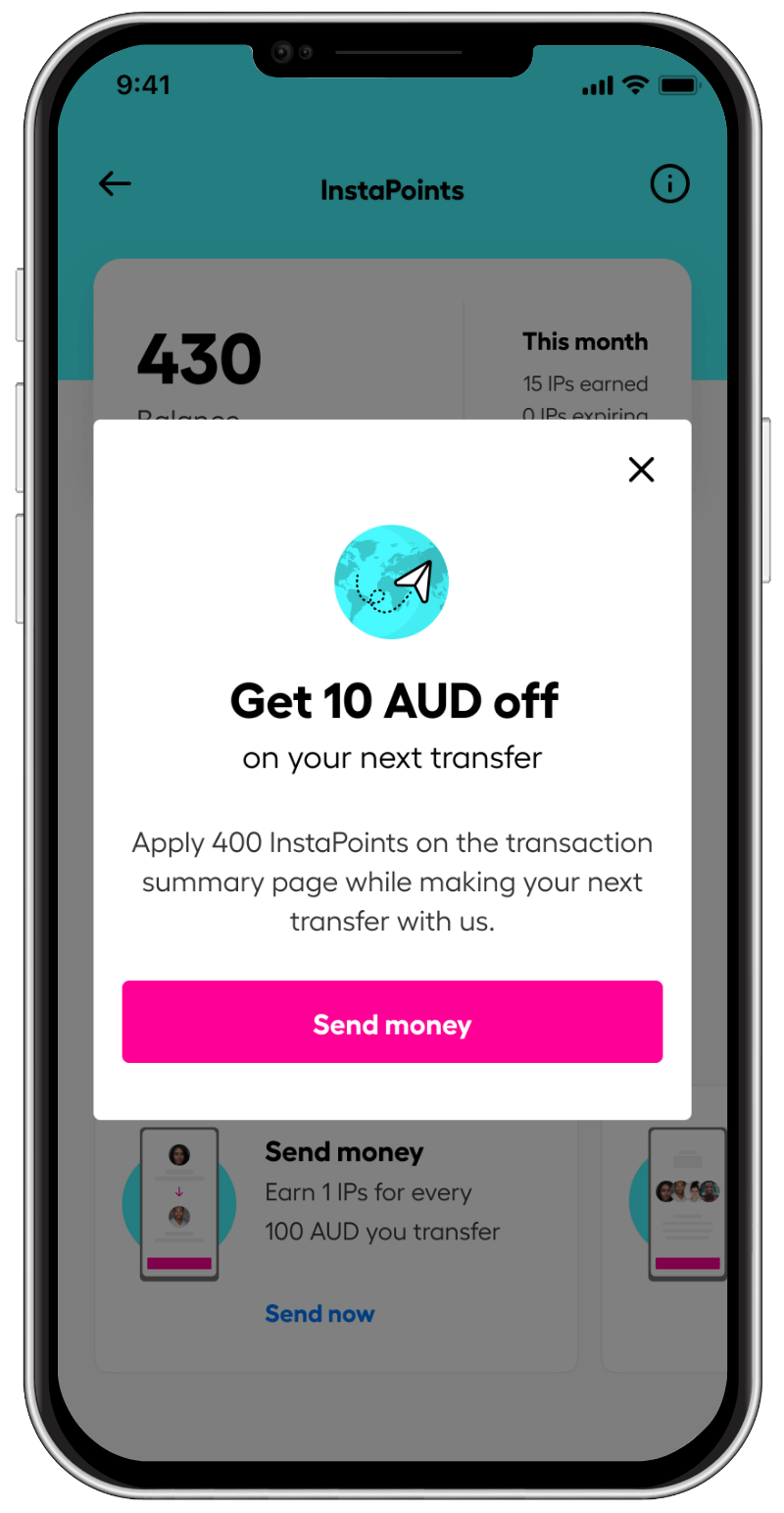Screenshot of a smartphone display at 9:41 AM showing full signal, WiFi, and battery icons. The screen highlights an application with a blue header at the top and a white background in the middle. The user has earned 15 points and is currently earning 1 point for every 100 AUD transferred. A USB text prompt suggests sending a message now. The interface features an arrow pointing down and a pink rectangle. The next section teases another smartphone, indicating a potential future feature or offer. A message states that the user will receive 10 AUD on their next transfer. The overall color theme of the app is predominantly white, pink, and blue.